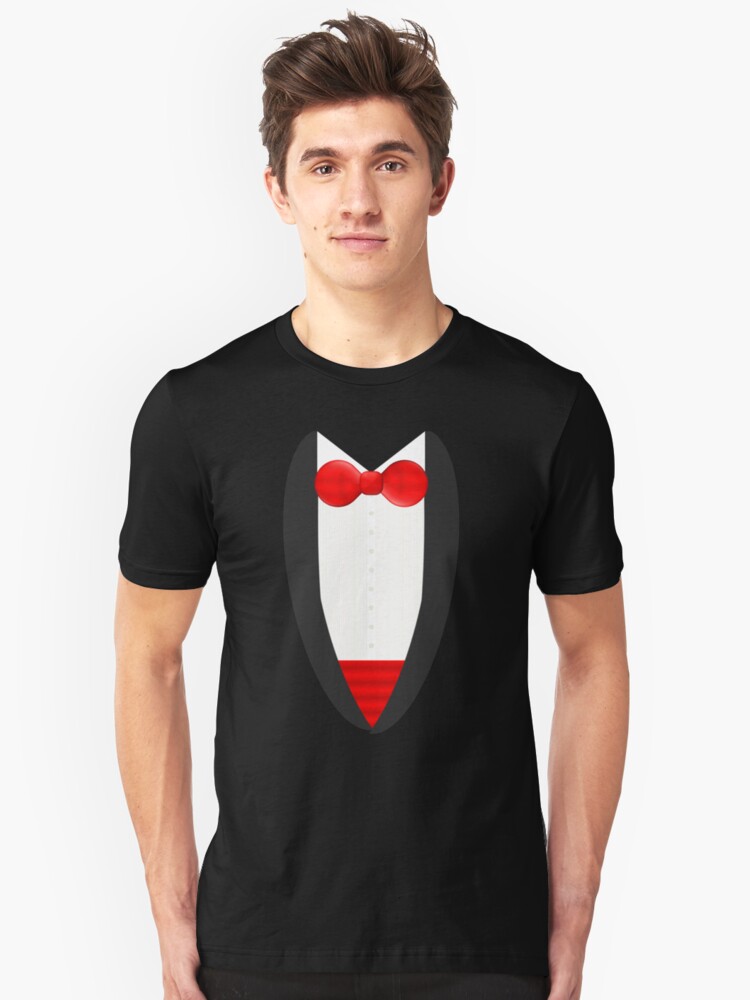The image features a young, white male in his 20s, staring at the camera with a light gray rectangular background behind him. He has dark brown hair that is medium in volume and stylishly combed up and back from his forehead, matching his dark brown eyebrows. He has brown eyes and a slightly forced smile on his face. 

He is wearing a short-sleeved, black, crew neck t-shirt that fits snugly against his arms, revealing his muscles. The t-shirt has a humorous tuxedo design printed on the front, featuring a red bow tie at the collar area and a white section resembling a dress shirt with black lapels on either side. Beneath the white 'shirt' is a red belt-like stripe near the waist. His arms hang straight down, with his hands positioned on his hips. The image is framed to show him from the top of his head to just below his waist, capturing his entire torso and part of his upper thighs.